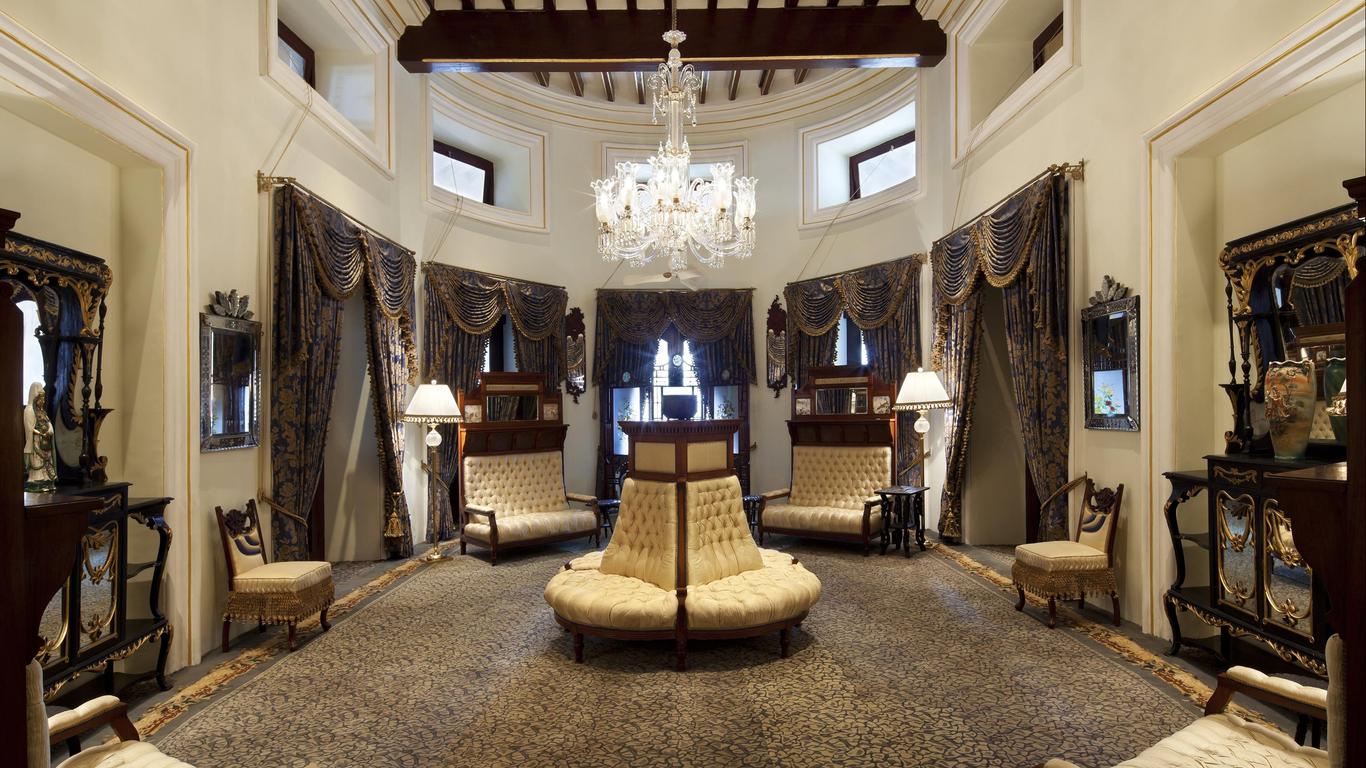This image depicts an opulent, highly detailed Victorian-style room, reminiscent of a stately home or a grand room in the White House. The room features an elegant, curved layout, lined with deep windows and heavy, intricate, brown and yellow drapes. There are five such windows, contributing to the room's bright yet regal ambiance. The centerpiece is an exquisite, large glass chandelier that hangs majestically from the ceiling, illuminating the room with a soft, luxurious glow.

The décor includes symmetrical arrangements of broad, cushioned chairs with tan upholstery and dark brown wooden frames, arranged low to the ground. These chairs are positioned along the walls and around the central circular seating area, emphasizing the optical symmetry of the space. Alongside the seating, two cabinets or armoires at the sides of the room display expensive-looking vases and possibly other artifacts, adding to the room’s affluent atmosphere.

Mirrors hang above the chairs on opposite walls, amplifying the room's spacious feel and symmetry. Detailed rugs with complex patterns cover the brown floors, adding another layer of sophistication to the surroundings. Additionally, two ornate lamps, featuring delicate crystals, flank the seating areas. The room also has two doorway entrances draped with similar curtains, providing access and adding to its grandiose sense.

This richly furnished space, with its asymmetrical yet meticulously balanced décor, possibly exists within a high-end museum or a palatial home, exuding an old-world, Victorian charm with meticulous attention to detail and style.